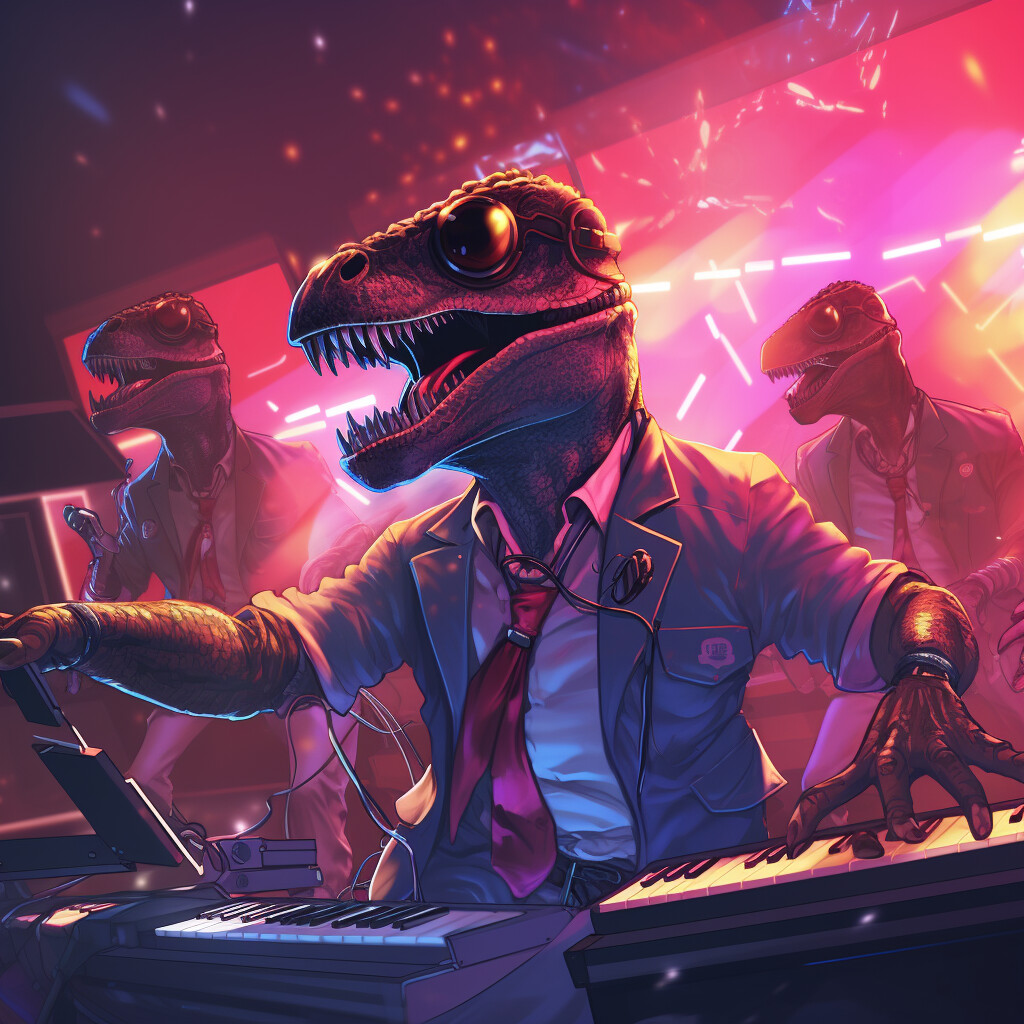In this computer-generated image, capturing a scene from a video game, we see three anthropomorphic dinosaurs dressed in modern-day attire, including gray suits, white shirts, and loose reddish ties. The central figure, a musician dinosaur, is prominently displayed in profile, playing two keyboards with its left dinosaur claw, while its right claw is extended upward, possibly holding a monitor-like device. This dinosaur has a wide, open mouth, revealing teeth and tongue, and a notably large, gold eye. Positioned behind this focal creature are two other humanoid dinosaurs, similarly attired, standing and facing west. The background is illuminated with multicolored lights in shades of reds and purples, resembling a concert or party scene.